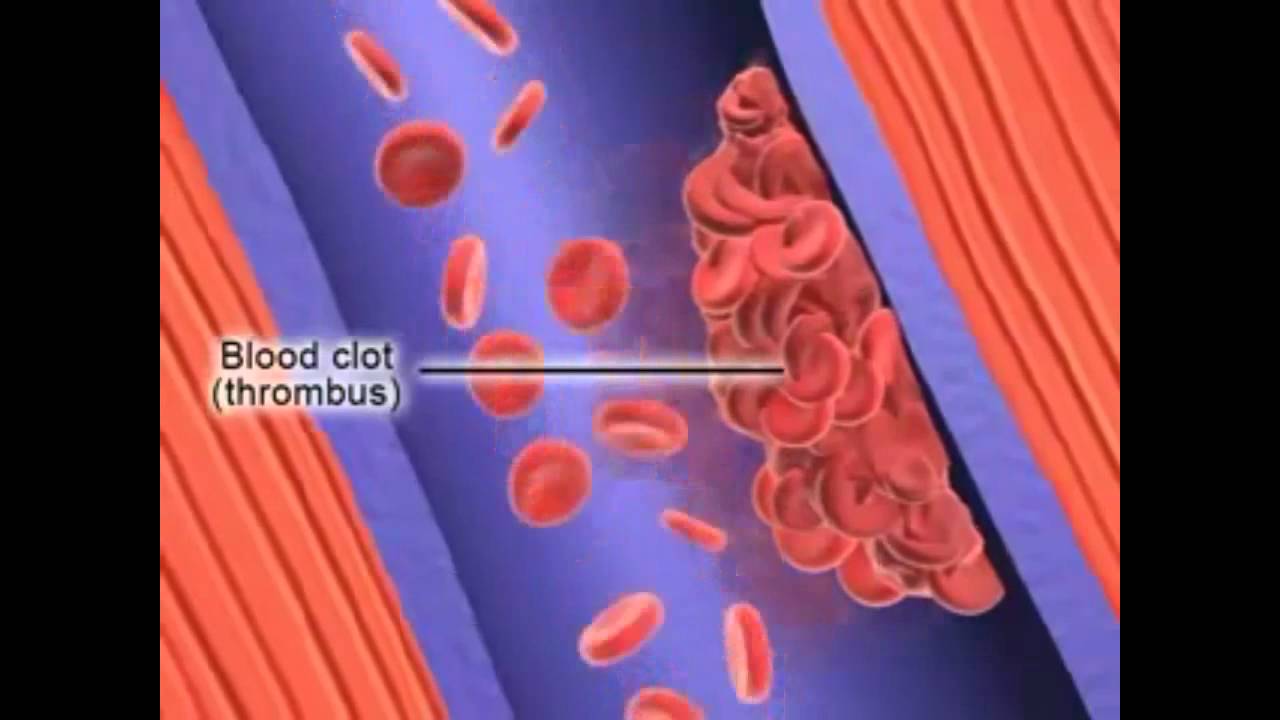This professionally illustrated diagram, potentially from a biology or medical textbook, depicts the formation of a blood clot within a blood vessel. Against a blue backdrop indicative of a vein, numerous red blood cells, which appear as small disk-like structures, float freely. Centrally, a significant cluster of these red blood cells forms a blood clot, labeled "blood clot thrombus" in parentheses. The image features distinct colors including black, white, blue, dark purple, gray, and reddish-pink, enhancing its detail. On the lower left and upper right, the image transitions to red-shaded areas, possibly representing muscle tissue surrounding the vein. There are black borders on the left and right sides of the image, but not on the top or bottom, hinting that this might be a screenshot from a video. The overall layout provides a clear and detailed illustration of a thrombus within the human body.